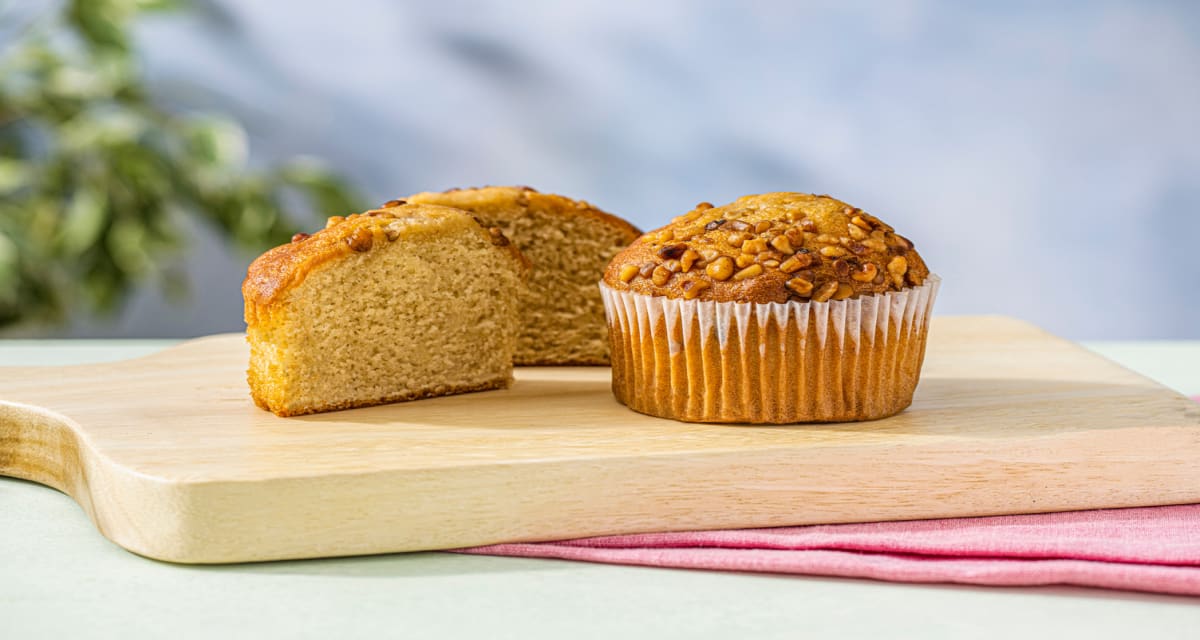A wooden cutting board, featuring a light wood color, sits atop a pink fabric napkin, which in turn is placed on a white table. Centered on the cutting board are two tan-brown muffins. One muffin remains wrapped in its paper muffin cup, while the other is cut in half, revealing a moist, off-white inner texture. The muffins are topped with either nuts or oatmeal, adding texture to their tops. The background is blurred and predominantly gray, with a hint of green foliage in the left corner, casting a subtle shadow. The entire setup is likely photographed in a kitchen setting, with the image presented in a horizontal orientation.